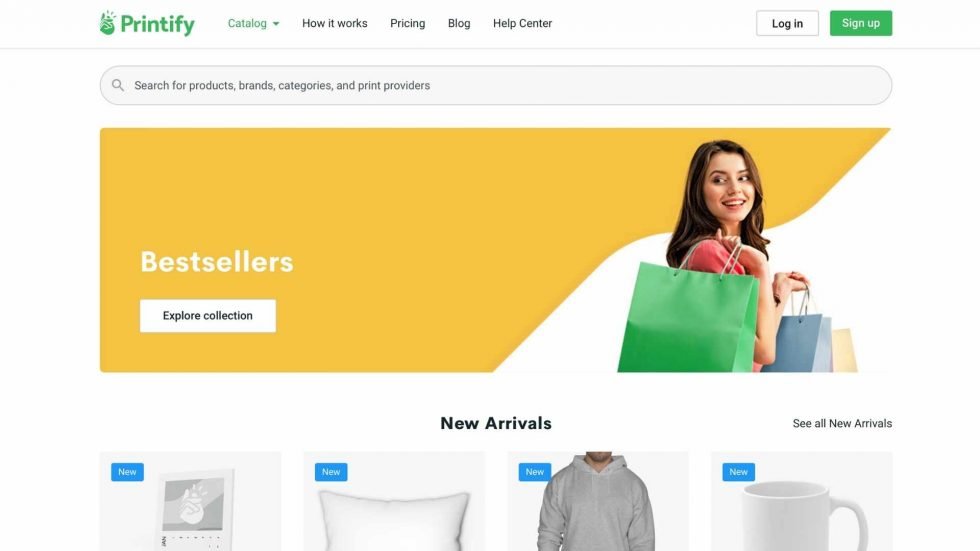This is a detailed caption for an image of a webpage from the Printify website:

---

The image captures a webpage from the Printify website. In the upper left corner, "Printify" is prominently displayed in bold green text, accompanied by a small, indistinct Printify logo. To the right of this, the top navigation bar includes several links: "Catalog," "How It Works," "Pricing," "Blog," and "Help Center," arranged from left to right. On the far right of the navigation bar are two buttons – a white "Log In" button and a green "Sign Up" button with white text. Beneath this navigation menu is a thin gray horizontal line spanning the width of the page.

Below this line, a long, gray search bar is centered, inscribed with "Search for Products, Brands, Categories, and Print Providers" in muted gray text. Further down, an image dominates the width of the screen. It features a woman captured from a side profile with her head turned toward the camera. She has long brown hair and is dressed in a pink short-sleeved top. In her hands, she carries multiple shopping bags in solid colors – pink, blue, and green. The backdrop splits into two sections: the area occupying about two-thirds of the screen is gold, while a white background frames the woman's body, creating a stark contrast. Her head, however, still lies within the gold section. 

On the left side of the image, bold white letters spell out "Best Sellers." Directly beneath this, a white button with the text "Explore Collection" in small black print invites further exploration.

---

This caption provides a comprehensive and detailed description of the webpage, highlighting both the graphical elements and the layout.